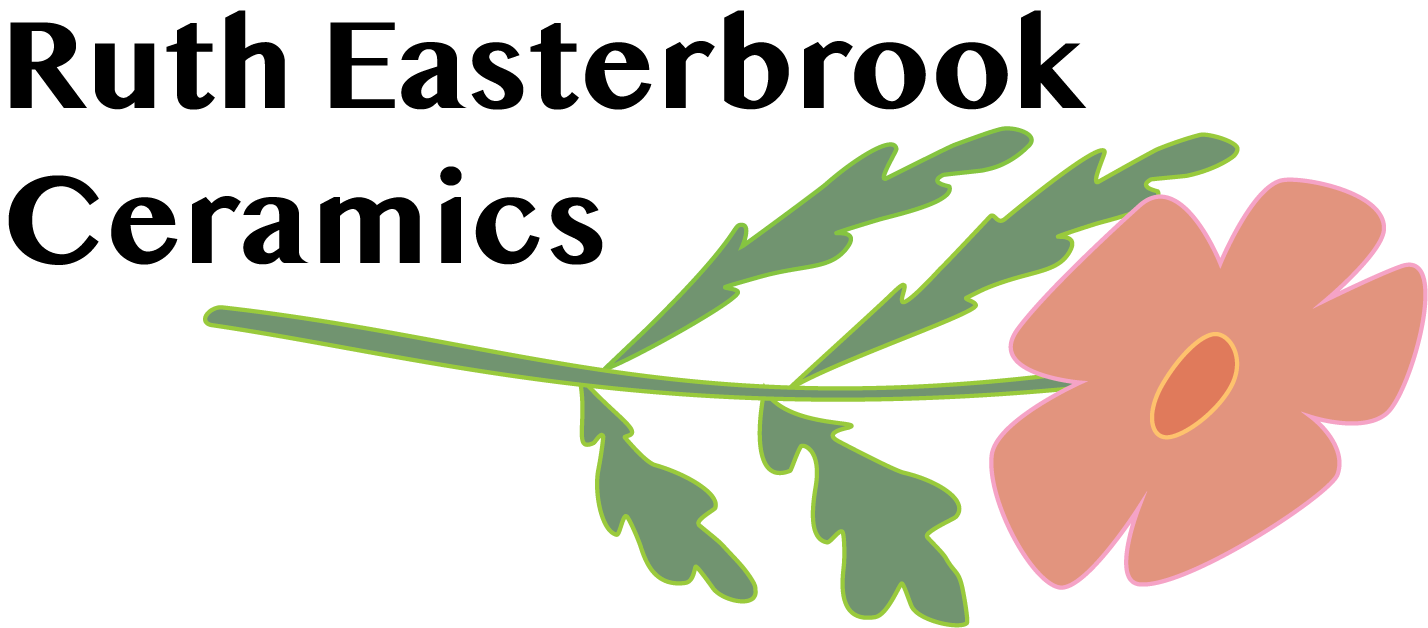The image features a horizontally laid, digitally drawn flower with five pink petals and an oval-shaped dark pink center, accentuated by a gold border. The flower has a green stem and four green leaves. This delicate flower, resembling a rose, is set against a solid white background, which takes up most of the image space. Two lines of black text are positioned in the upper left corner, reading "Ruth Easterbrook Ceramics." The simplicity and elegance of the design make it a striking and understated visual.